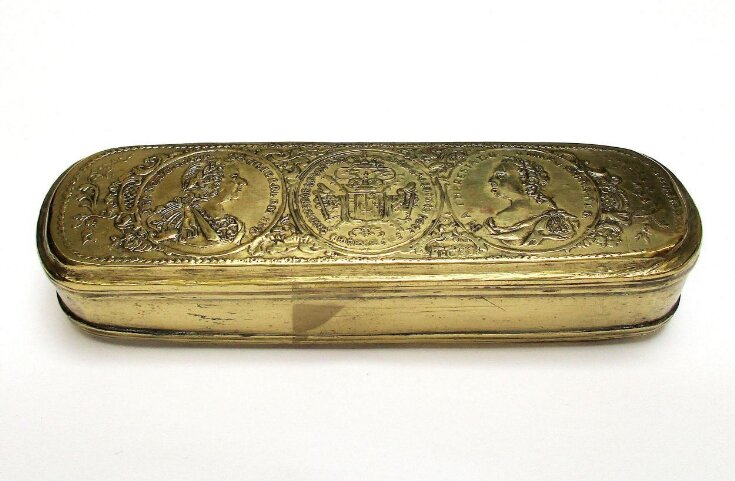This image showcases an oblong-shaped, antique brass box with a long-rounded rectangular form. The box appears to be thin and rests on a white table, where its reflection and some wear-induced scratches on the right side are visible. The lid of the box features an ornate, raised decorative motif characterized by three equally spaced circular elements. Each circle has a distinct feature: the far-left circle presents the profile of a man with curly hair, while the far-right circle depicts the profile of a woman, also with curly hair, and adorning a gown. The central circle seems to contain a coat of arms or a seal, likely suggesting some Roman or Greek influence. These circles are reminiscent of coins approximately the size of a quarter and are surrounded by intricate filigree designs, enhancing the box's antique charm.